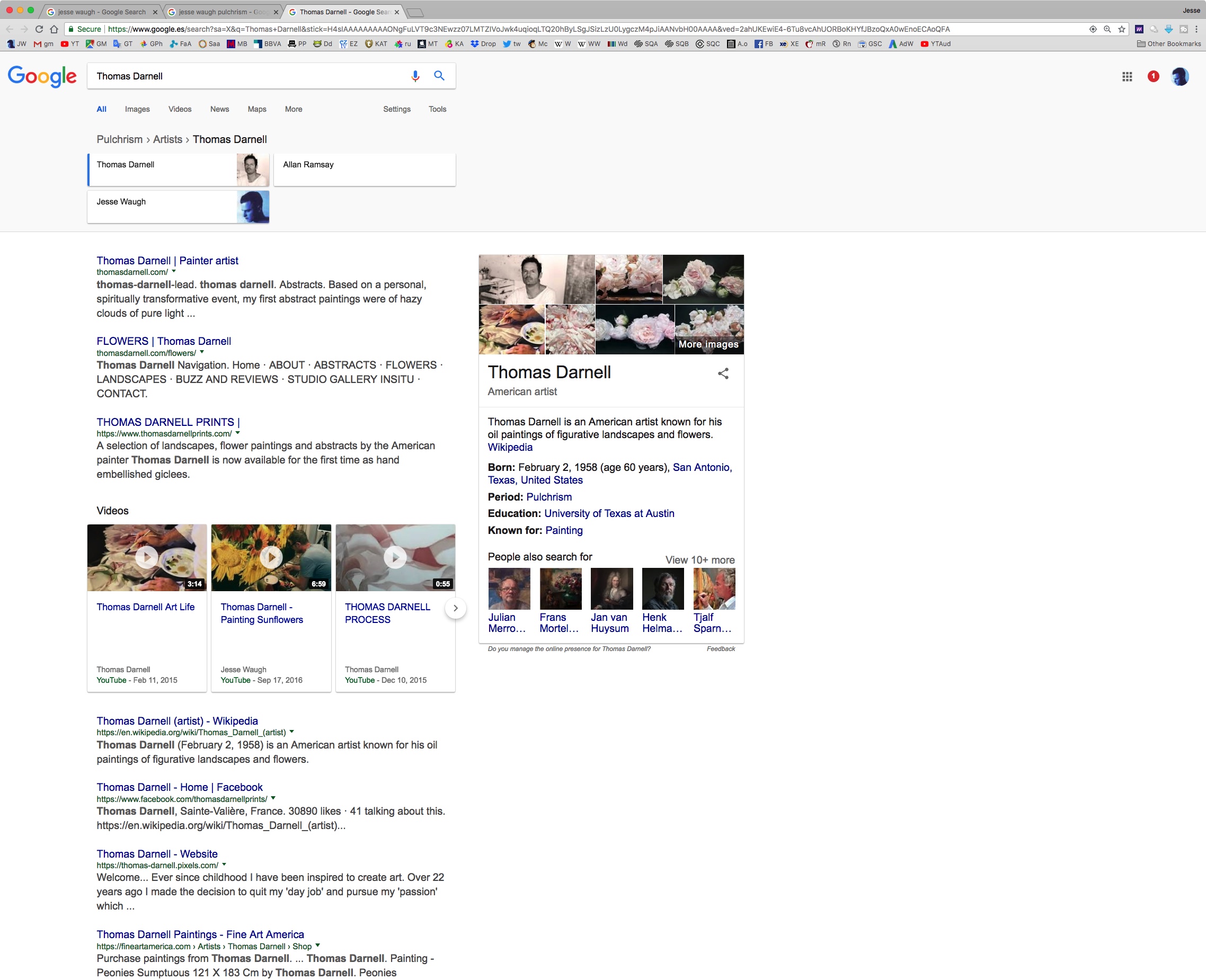The image depicts a Google search results page with three tabs open on a browser running on an Apple device, as indicated by the characteristic three dots at the top of the screen. The search query entered is "Thomas Darnell," an artist. 

At the top of the page, to the left of the search bar, the Google logo is displayed, while to the right, options for voice search and a magnifying glass icon for search are visible. The "All" tab is highlighted in blue, indicating it is the current selection, with other tabs including Images, Videos, News, Maps, and More available.

Below the search bar, Google suggests related topics such as "Pulcherism" and "Artist," alongside a right arrow leading to additional topics for Thomas Darnell. A brief profile of Thomas Darnell appears first, with a thumbnail image of him displayed. Other notable mentions include Alan Ramsey, listed without an accompanying image, and Jesse Wah, positioned right under Thomas Darnell.

The search results include various types of content. Initially, there are links to websites providing further information about Thomas Darnell. Each link is presented with the website title, the URL in green, and a brief description of the page content. Among these are pages dedicated to his flower-themed artworks and Thomas Darnell prints. 

Following the initial web links, there are three YouTube videos related to Thomas Darnell, each noted with their upload dates. Additional website links appear further down, continuing to offer more extensive information about the artist.

On the right-hand side of the search results, there's an information box with multiple images of Thomas Darnell's works, providing an option to see more images. A concise Wikipedia excerpt is also included, detailing his birthdate as February 2, 1958, and briefly outlining his background as an American artist known for his oil paintings.